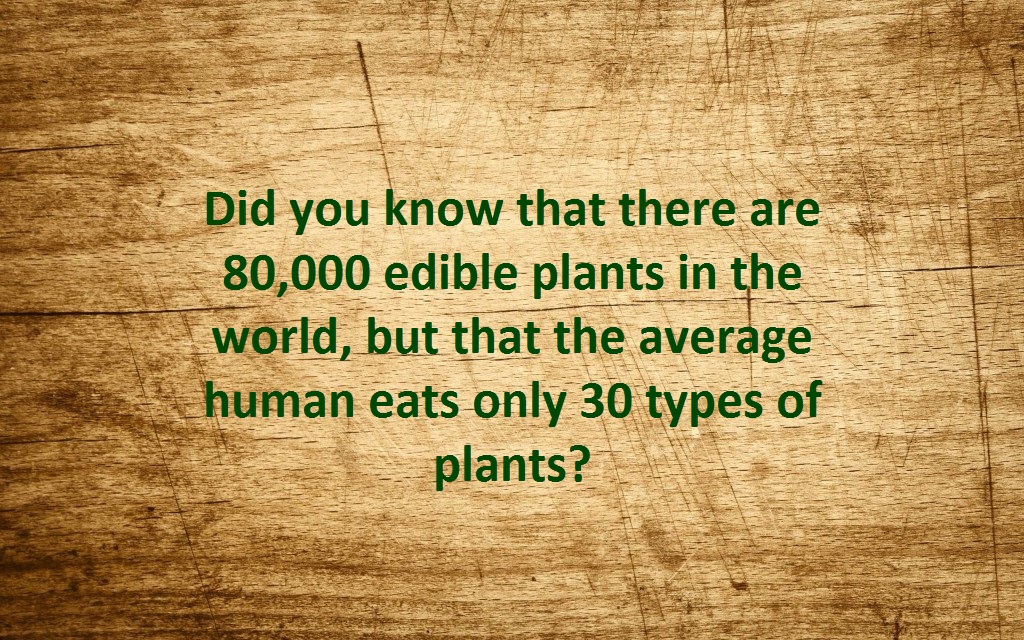The image is a rectangular photograph with the width being greater than the height. It features a wooden surface background that appears to have numerous scratches and knife marks, reminiscent of a well-used cutting board. The wood varies in color, being a darker brown near the edges and transitioning to a lighter brown towards the center.

At the center of the image, text is prominently displayed in green font, which reads: "Did you know that there are 80,000 edible plants in the world? But that the average human only eats 30 types of plants?" This fun fact highlights the diversity of edible plants compared to the limited variety typically consumed by humans. The text is well-centered and is not embedded on either side of the image, standing out clearly against the textured wooden background.